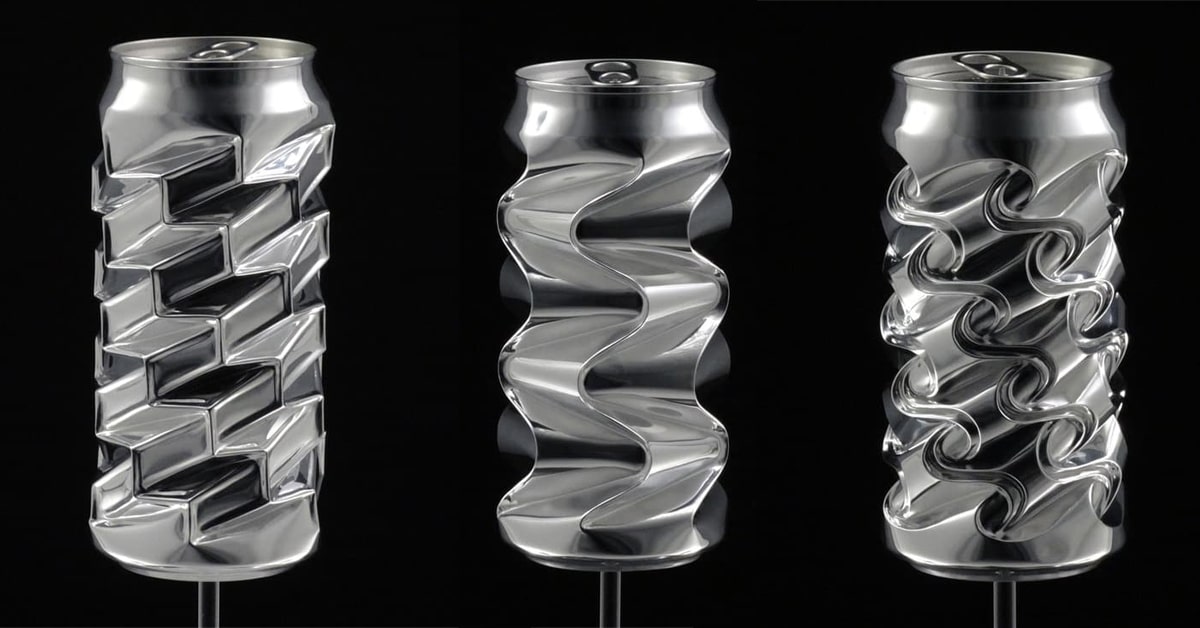The photograph showcases a striking display of three artistically modified silver soda cans set against a black background, each perched atop slender metal poles. These cans retain their traditional pull tabs and rims, but their bodies are intricately transformed with distinct geometric patterns. The leftmost can features a series of step-like structures forming a 3D, stair-step effect encircling its surface. The middle can is adorned with wavy, ribbon-like patterns that elegantly swirl around its form. The can on the right boasts a design reminiscent of interlocking strands or a DNA helix, with repeating 'S' shapes weaving diagonally across its side. This artistic arrangement highlights the malleability of the metal and showcases each unique pattern in a cohesive, eye-catching presentation.